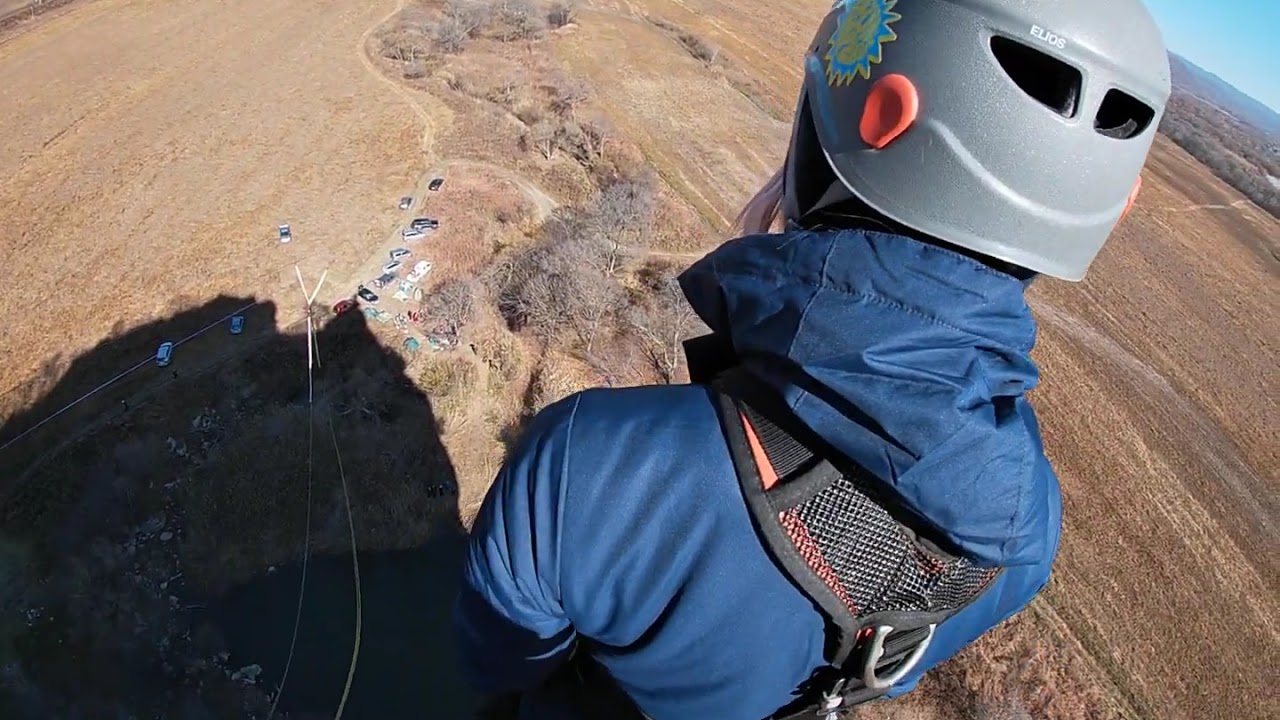In this photograph, a female climber stands atop a towering, rugged cliff, her back turned to the camera as she gazes down at the sweeping landscape below. She wears a dark bluish-green windbreaker and a distinctive gray climbing helmet adorned with a blue and yellow sun logo. Her pinkish hair peeks out from beneath the helmet, adding a splash of color to her gear. A black mesh harness with orange accents and silver clips wraps snugly around her, prepared for any daring feats. The vast drop below her reveals distant fields and a sandy patch with a parking lot, where tiny cars hint at the enormous height she's scaled. The scene is bathed in the bright light of a clear, sunny day, highlighting the climber's adventurous spirit and the breathtaking view she commands.